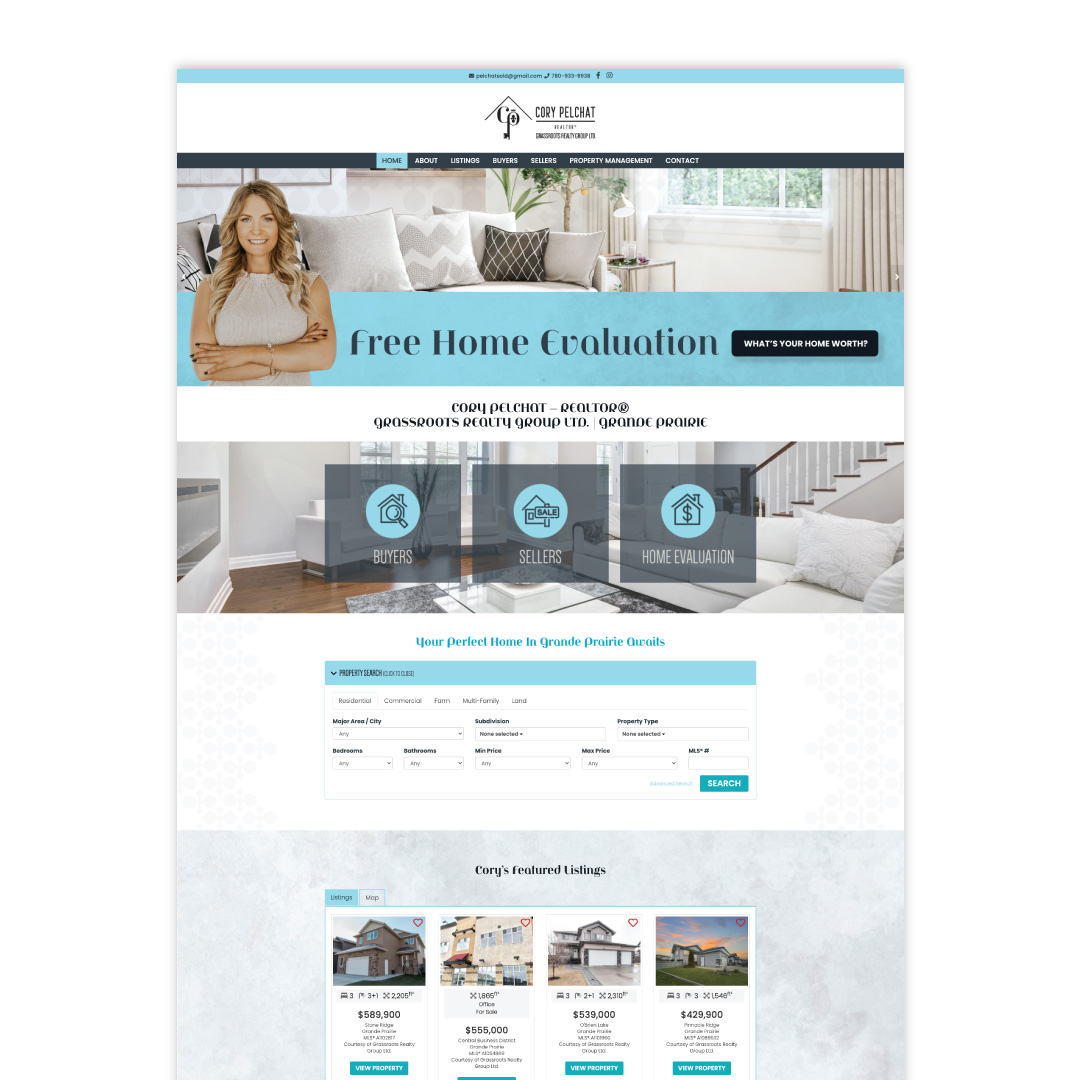In the screenshot of the website, prominently titled "Cori Peel Chat" at the top center, we observe a well-organized real estate platform. The navigation menu at the top of the page includes tabs for "Home," "About," "Listings," "Buyers," "Sellers," "Property Management," and "Contact," offering easy access to different sections. 

On the left side, there is a photo of a woman, presumably Cori Peel. Central to the page is a highlighted feature stating "Free Home Evaluation," accompanied by a call-to-action button on the right labeled "What's Your Home Worth?". Below this, further information designates Cori Peel as a Realtor affiliated with Grassroots Realty Group in Grande Prairie.

The website also includes three prominent buttons in a subsequent section for "Buyers," "Sellers," and "Home Evaluation." Accompanying these is a form titled "Your Perfect Home in Grande Prairie," providing various text boxes and drop-down menus for users to fill out their details.

Towards the bottom of the page, there is a segment labeled "Cori's Featured Listings," showcasing four different properties. Each listing is displayed with a photo of the property’s exterior, some brief details, and a "View Property" button for more information.